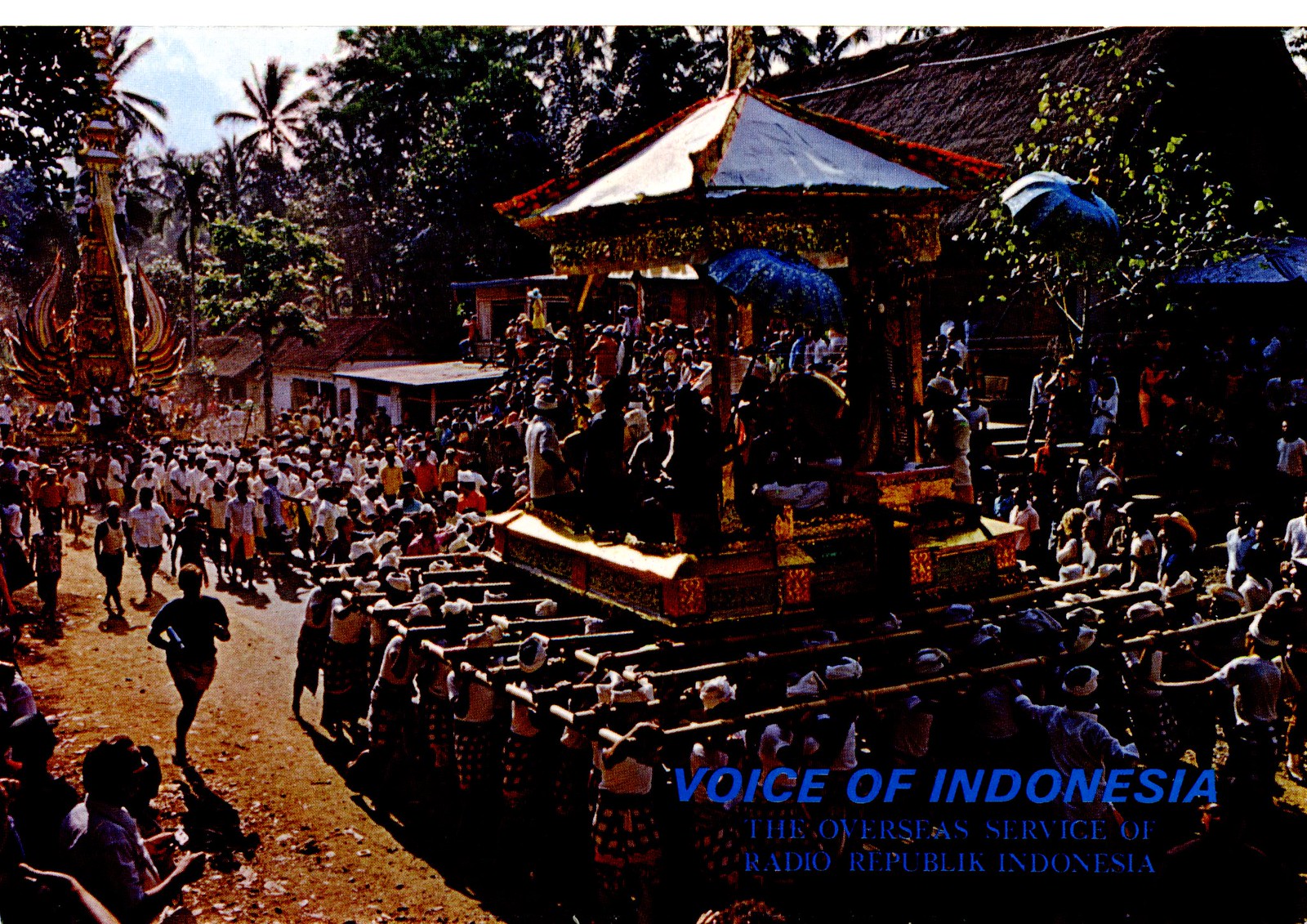In this heavily contrasted and edited photo, a large crowd is depicted in the midst of a vibrant festival or parade. Central to the image is a substantial group of about 50 people carrying a structure resembling a small gazebo or mini temple on their shoulders, supported by long beams or bars. Seated within this elevated structure are likely important figures, perhaps of royal or noble status. Engulfing this scene is a massive sea of people, both participants and onlookers, contributing to the festive, celebratory atmosphere. Additionally, in the distant background on the left, there's a float or possibly a Hindu temple that adds to the cultural richness of the procession. Notably, in the bottom right corner, blue italicized and capitalized text reads "Voice of Indonesia, the Overseas Service of Radio Republic Indonesia."